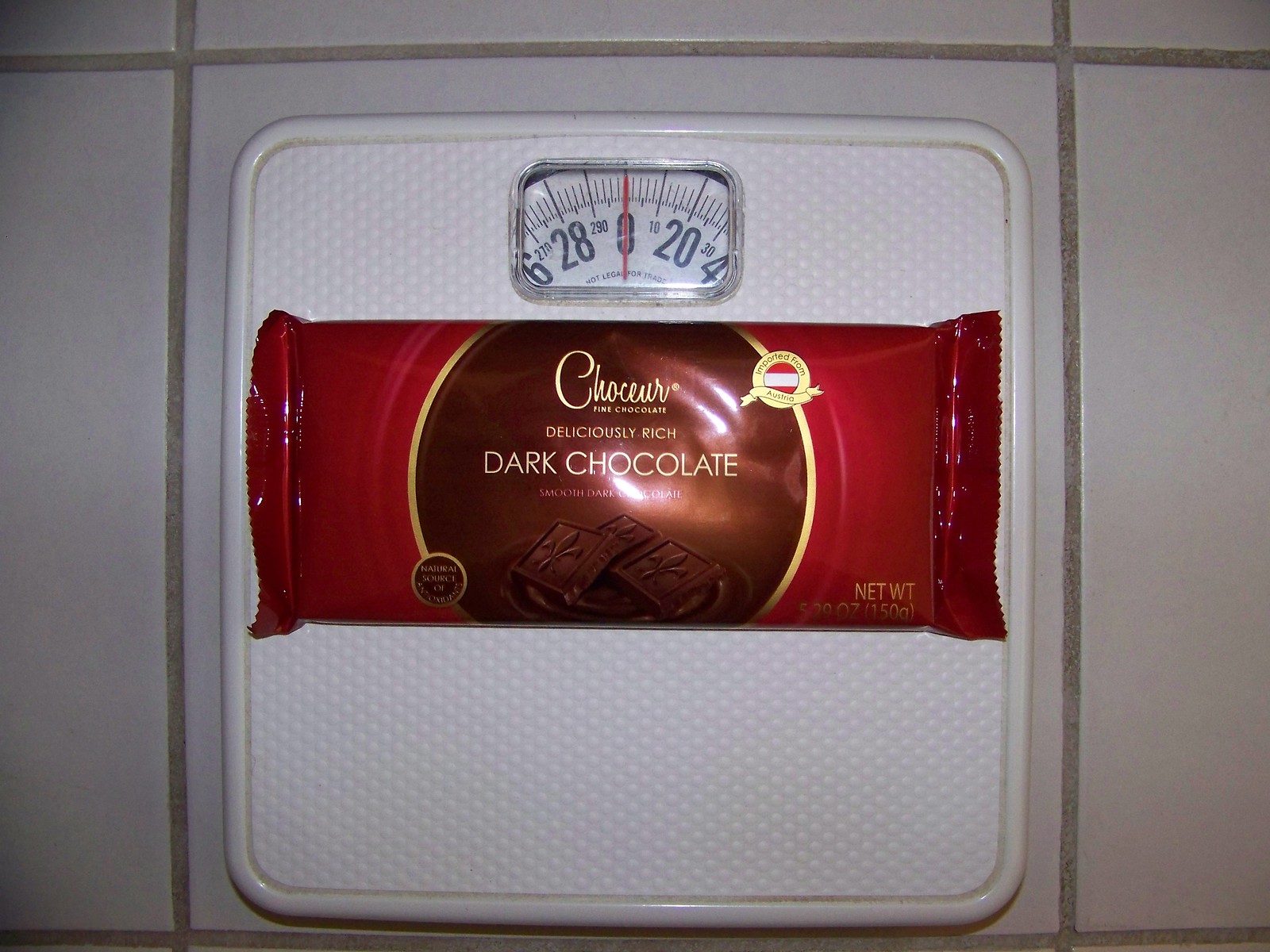In the image, a white scale sits on grayish-white tile with gray grout. Atop the scale is a packet of dark chocolate, wrapped in predominantly red packaging with a brown circular area in the center showcasing an image of the chocolate. The brand name appears in a cursive font that's difficult to read but seems to say "Choser" or something similar. The packaging touts various descriptions including "fine chocolate," "deliciously rich dark chocolate," and "smooth dark chocolate." The chocolate squares depicted on the packet feature an intricate pattern. Despite the package resting on the scale, the scale's display reads zero, suggesting that the weight does not register, perhaps because the package is relatively light, around 150 grams. An additional detail includes a label indicating the chocolate is "imported from Austria," accompanied by an Austrian flag.